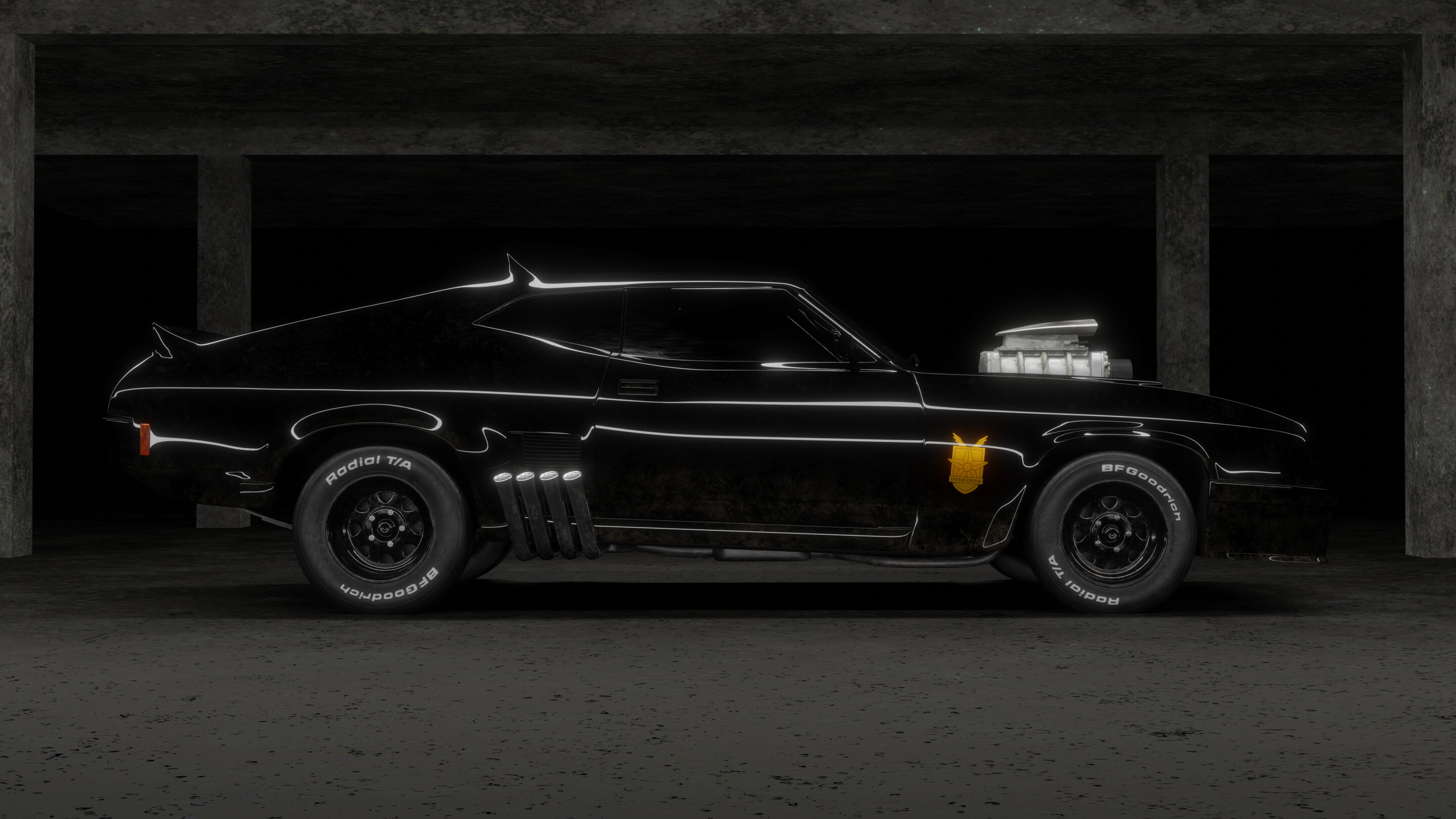Here is a detailed, cleaned-up caption:

"This striking 1967 Black Dodge Charger showcases an intimidating presence with its BF Goodrich Radial T/A tires, featuring iconic white lettering on their black walls. A gold crest adorns the back of the front fender, adding a touch of elegance to its muscular exterior. The muscle car boasts a distinctive four-outlet exhaust system, with gleaming chrome pipes that promise a powerful roar. Tinted windows add a touch of mystery, while the turbocharged engine, prominently visible through the custom hood, hints at its performance pedigree. Enhanced aerodynamics come from the rear spoiler and an additional spoiler mounted on the roof, underscoring its readiness for high-speed street racing. This meticulously maintained Black Dodge Charger epitomizes the spirit of a true street racer’s dream ride."